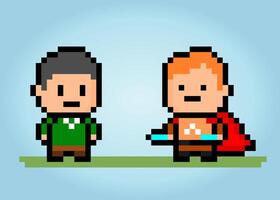This image is a vintage-style 8-bit cartoon illustration reminiscent of early video game graphics. It features two pixelated male characters with light peach-colored skin standing side by side on a green strip of grass against a plain blue background. The character on the right has reddish-orange hair, wears an orange shirt, a distinctive red cape, and holds two blue items in his hands, possibly resembling weapons or tools. The character on the left has dark gray, almost black hair, a green long-sleeved shirt, and brown pants. Both characters have simplistic square eyes and long rectangular mouths, capturing the classic pixelated aesthetic.